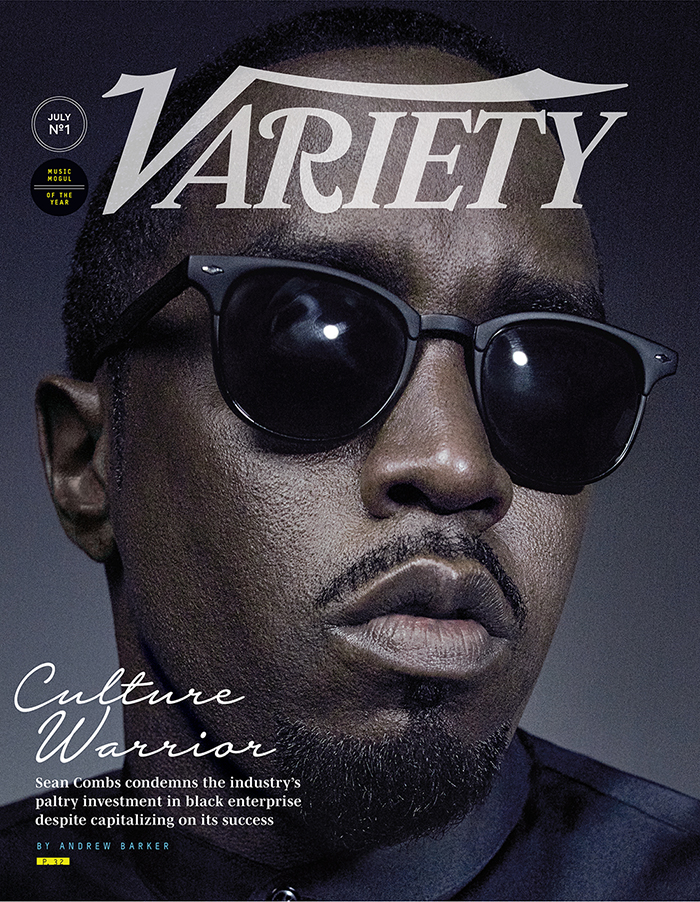The cover of Variety magazine's July issue features an intense and detailed close-up of Sean Combs, also known as Puff Daddy or P. Diddy, taking up nearly the entire page. His serious visage stems from his dark sunglasses with black lenses reflecting the photographer's lights. He has a short, neatly trimmed goatee and mustache, with meticulously groomed short black hair, lightly flecked with white, indicating his age. Above his forehead, the magazine's name, "Variety," is emblazoned in bold white letters. In the top left corner, enclosed in circles, it reads "July 1" and "Music Mogul of the Year." The bottom left corner highlights a compelling feature titled "Culture Warrior," with a subtitle reading, "Sean Combs condemns the industry's paltry investment in black enterprise despite capitalizing on its success," written by Andrew Barker, directing readers to page 17. The backdrop is a subtle gradient gray, ensuring focus remains on Combs' striking and powerful image.